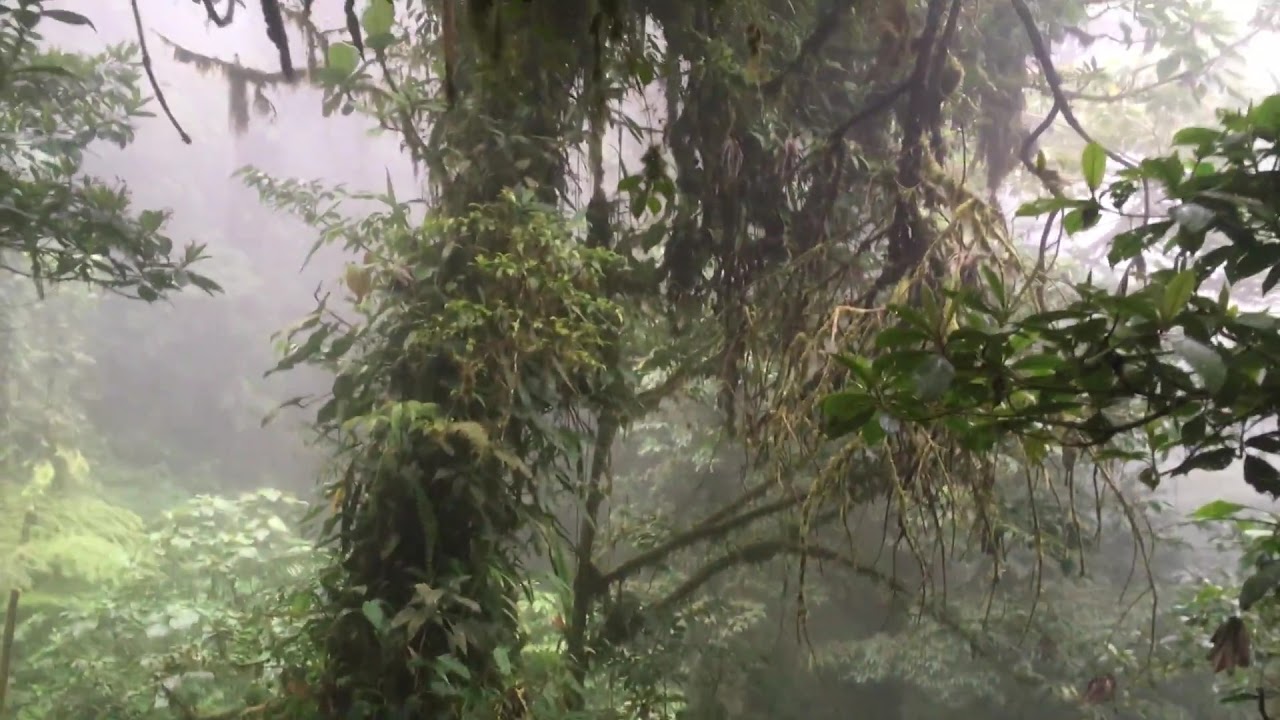A foggy, dense forest scene dominates this image, enveloped in an almost eerie mist that pervades the landscape. Towering evergreen trees, some not in the best condition, rise amidst a rich spectrum of greens from various bushes and grasses scattered throughout. The forest floor and lower branches exhibit hues of brown and black, while the thick fog adds layers of white and gray, creating a muted, mysterious atmosphere. A particularly large tree stands prominently in the middle, surrounded by smaller shrubs and branches flanking the sides and top, enhancing the chaotic harmony of nature. There are no objects or text in the image, drawing the focus solely to the wild, verdant expanse that seems to capture a moment in the middle of the day. The scene suggests a location that could be in a lush region, possibly in Central or South America or Asia.